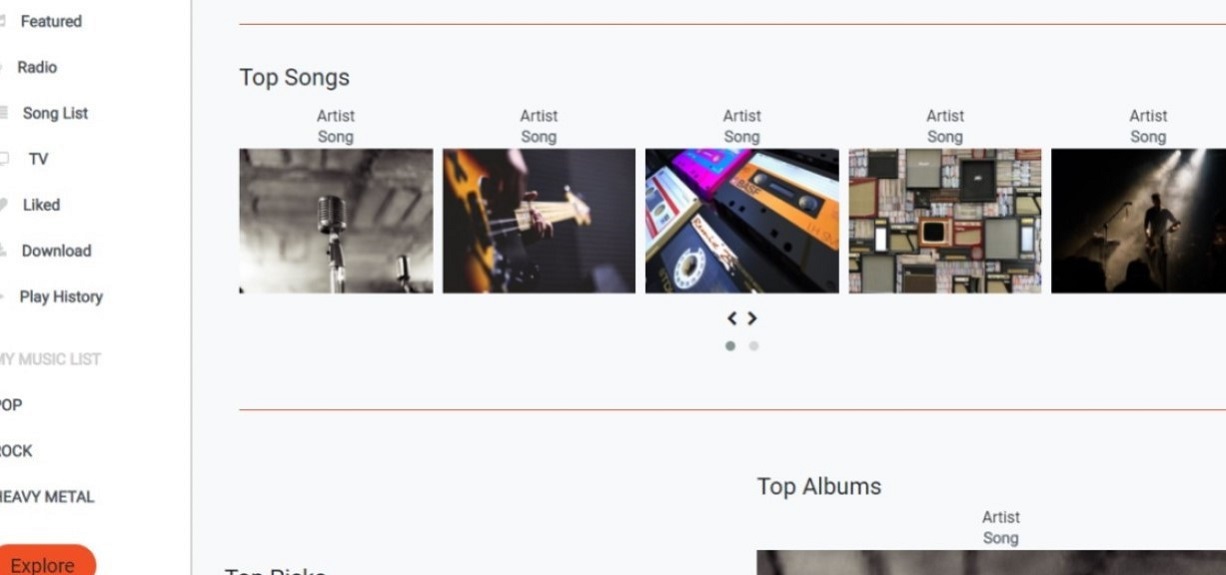The screenshot depicts a music-related interface featuring various categories and visual elements. At the top, a section labeled "Pop Songs" is visible, showcasing a grid of album covers. Each album is tagged as "artisong," which appears multiple times. Below this, another section titled "Top Albums" is highlighted, along with options such as "Feature," "Radio," "Song List," "TV," "Like," "Download," "Play History," "Music List," "Rock," and "Heavy Metal," among others, indicating the diverse music genres and functionalities available.

In the "artisong" category, the first album cover displays an image of a vinyl record. The second album cover features a performer on stage, capturing the energy of a live performance. The third album showcases four cassette tapes, evoking a sense of nostalgia. The fourth one presents three old-fashioned televisions, with the background TV showing a man playing a guitar, blending retro aesthetics with a musical theme.